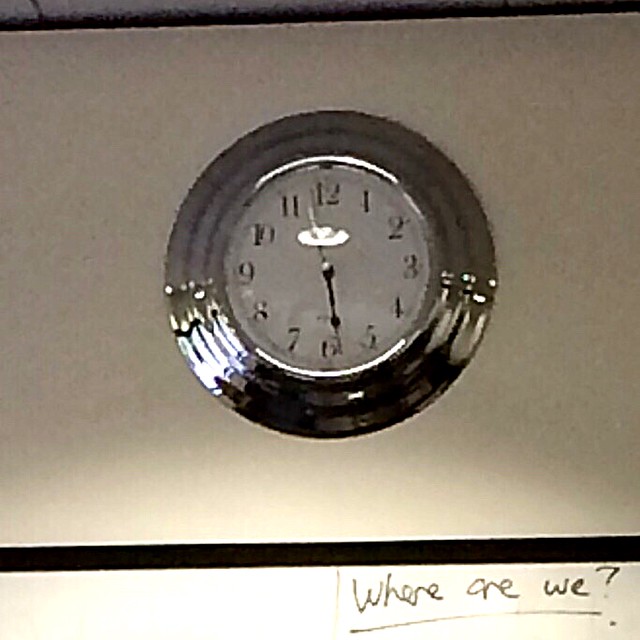The image depicts a grainy and noisy color photograph of a round analog wall clock mounted in the center of a cream-colored wall. The photograph, likely taken with a low-quality or old smartphone camera, is marred by patches of pink, green, and black streaks, indicating poor image quality. The wall clock, which has a shiny chrome bezel, features a white face with standard black numbers and reflective glass, showing the time at approximately 11:29, with the minute hand pointing near the six and the hour hand between 11 and 12.

Below the clock, a handwritten text in black reads "Where are we?" which is underlined. This text is placed on or near a whiteboard, suggesting the setting might be a school or educational environment. A horizontal black line spans the width of the image above the text. The wall’s coloring appears inconsistently due to the noise, showing shades of pinkish gray as well.